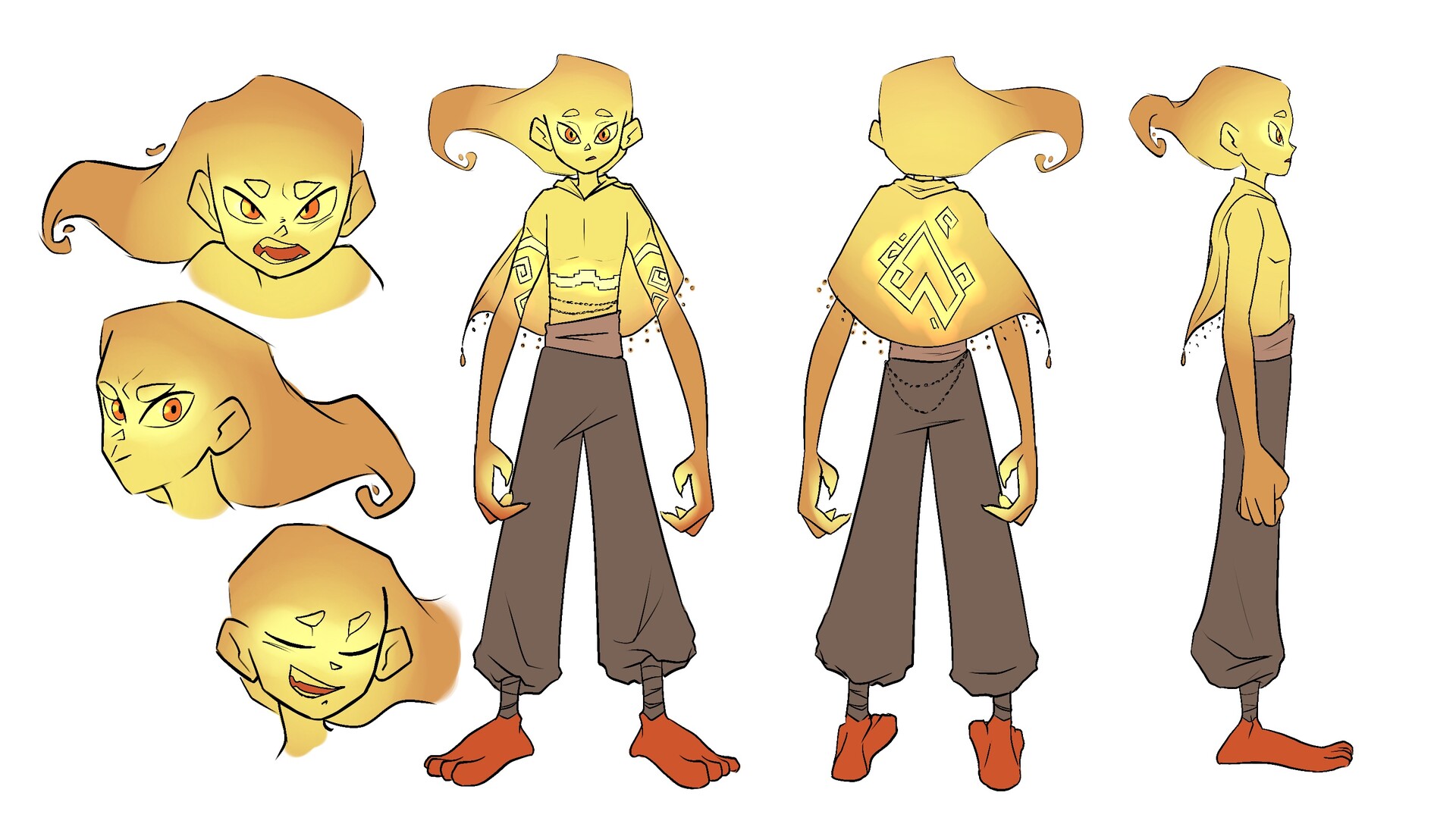This illustration features a detailed character design sheet against a solid white background, likely intended for a comic book or cartoon. The left side of the image depicts three vertical headshots capturing different expressions: at the top, the character looks mad; the middle head tilts slightly left and appears interested; the bottom head showcases a slight smile. The right side of the illustration presents three full-body images of the character from different angles: facing forward, with their back turned, and a right-facing profile. 

The character stands out with their distinctive appearance. They sport no shirt but have a small cape attached to their shoulders. Their body appears to glow, emanating a yellow light that fades into an orange hue at the extremities, including their flame-like hair. Adorning the upper arms and torso are simple geometric tattoos. The character wears a purple belt and baggy brown pants tied at the ankles, revealing big red feet with four visible toes. The character's eyes are a striking orange, adding a final touch to their unique and vivid design.